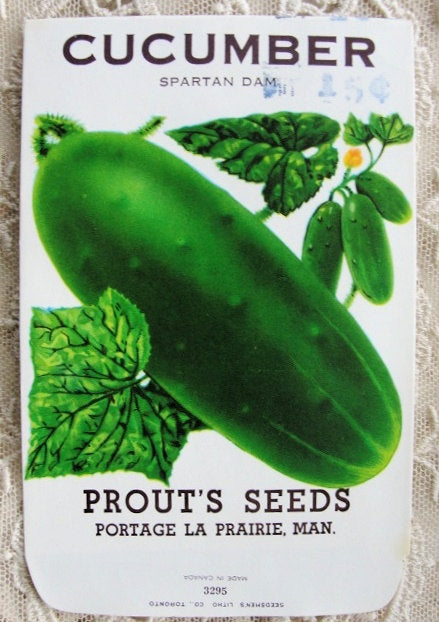This is a detailed photograph of a vertical seed packet resting on a table, which is adorned with a beautiful white lace tablecloth. The seed packet itself is white and prominently features a large image of a bright green cucumber oriented diagonally, surrounded by lush green foliage, including a few smaller cucumbers and a tiny yellow flower on the vine. The packet also depicts three additional cucumbers in the process of maturing. In bold black lettering at the top, it reads "Cucumber Spartan Dam," while the bottom of the packet bears the inscription "Crouch Seeds, Portage La Prairie Man." Additionally, there is some very small, light gray text at the bottom which is illegible. The overall design of the packet suggests it might be an older vintage, possibly from the 60s or 70s, and it could easily be mistaken for a label from a jar or an advertisement poster due to its detailed artwork and layout.